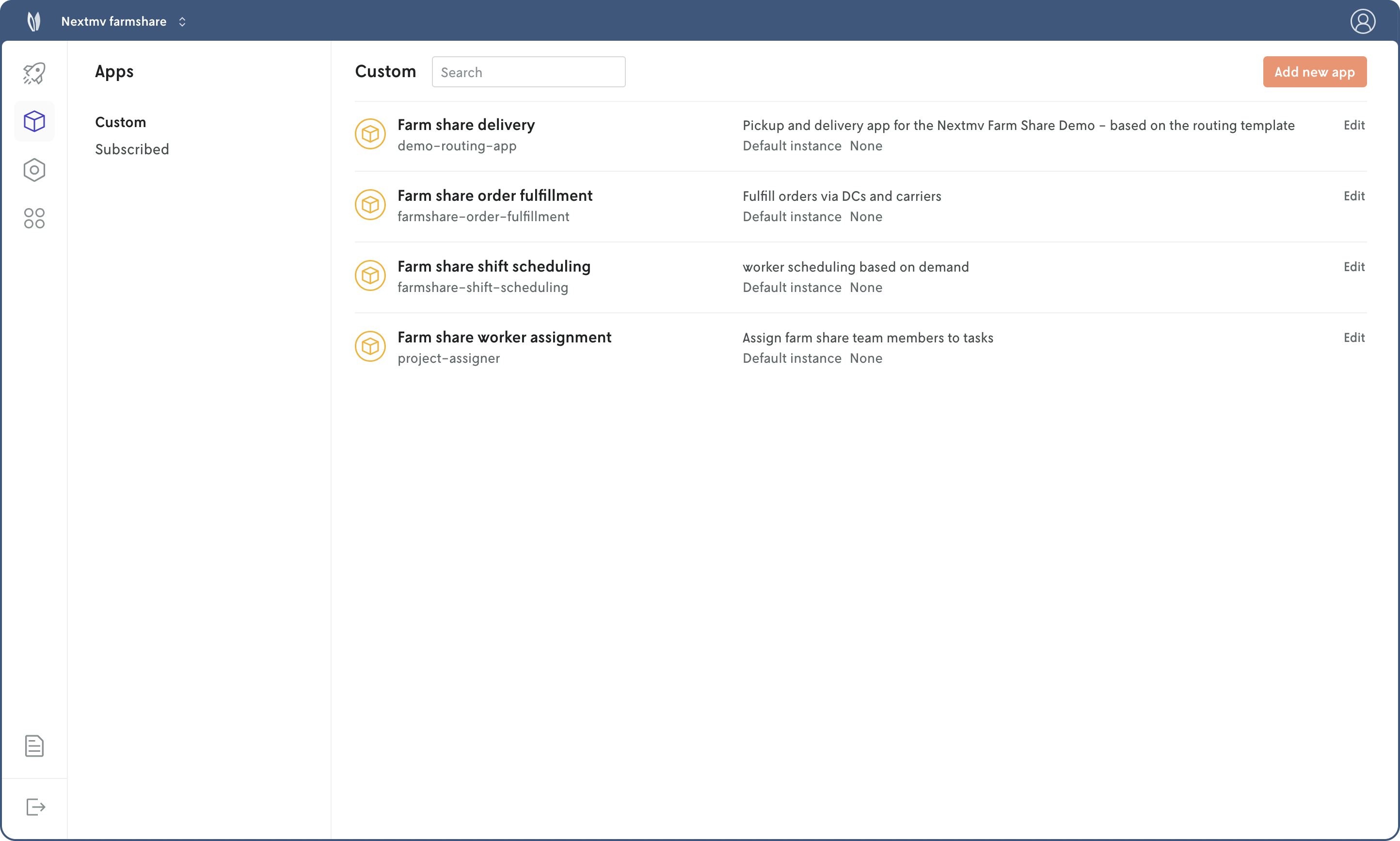In this image, we are viewing a screenshot of a software interface. The top header is a dark bluish-gray color featuring white text. On the left side of the header, a logo resembling two leaves carries the text "Next My Farm Share." In the upper-right corner, there's a circular icon with an individual's profile image. 

Below the header, on the left sidebar, the options labeled "Apps," "Custom," and "Subscribed" are visible. To the right of the sidebar, "Custom" is prominently displayed in bold black text, accompanied by a white search bar to its right. In the upper right of the main content area, an orange action button labeled "Add New App" stands out against the white background.

The central section of the interface lists several applications associated with "Farm Share" programs. The applications are: 
1. "Farm Share Delivery Demo Routing App"
2. "Farm Share Order Fulfillment"
3. "Farm Share Order Fulfillment" (appears twice)
4. "Farm Share Shift Scheduling"
5. "Farm Share Worker Assignment"

Below these listings, the interface displays the text "Project Assigner." Accompanying it is a description that reads, "Assign Farm Share Team Members to Tasks." 

Additionally, a section labeled "Default Instance" is also present, currently showing "None." 

The layout and structure of the interface are clearly organized to facilitate the management and customization of various farm share-related applications.